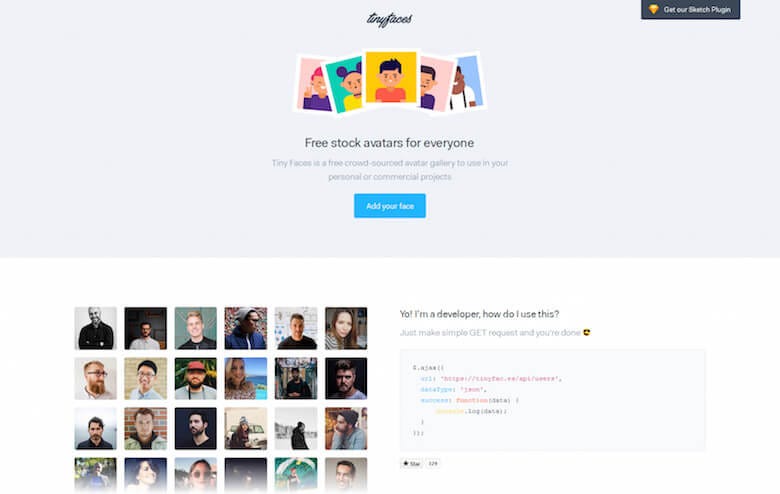The image showcases the interface of what appears to be a photo editing website focused on avatars. At the top of the image, centered, the title "Tiny Faces" is displayed in a cursive font. To the top right, there's a black box with white text that reads "Get Our Sketch Plugin."

Below the title, five small photos of people are aligned horizontally: a man, a woman, and three men in sequence. Under these thumbnails, the bold text "Free Stocks, Avatars for Everyone" is prominently displayed. Directly below this, in a lighter font, it states, "Tiny Faces is a free crowdsourced avatar gallery to use in your personal or commercial projects."

Further down, a light blue box with white text prompts users to "Add Your Face." At the bottom left corner of the image, several rows of photos are organized, each containing six avatar images arranged four rows down. In the first row, the avatars are five men followed by one woman. The second and third rows mirror each other with four men and two women. The final row features two women among four men, set in a varied sequence.